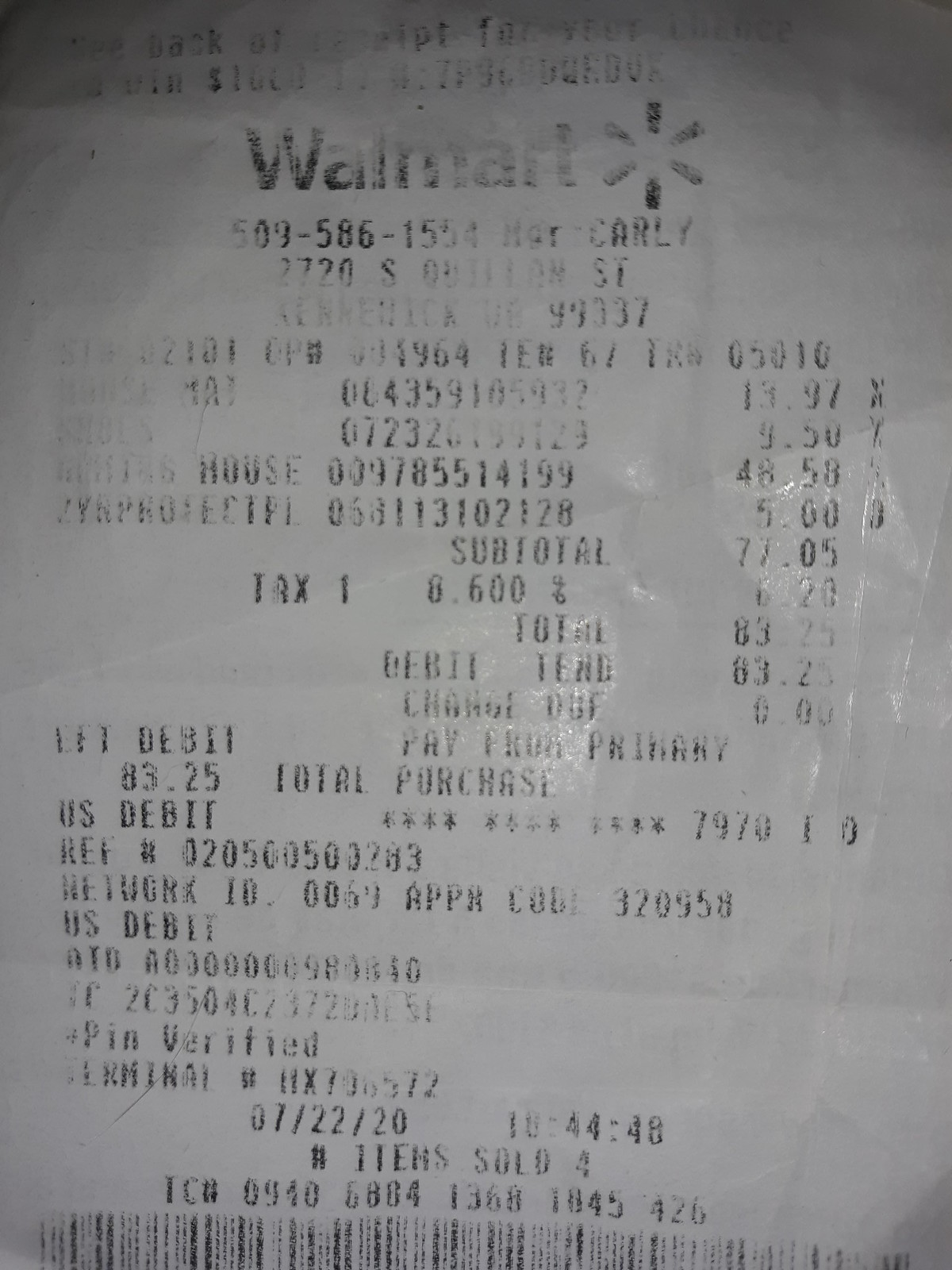This image captures a faded and slightly wrinkled Walmart receipt. At the top, the Walmart logo is visible with the signature Walmart star beside it, followed by some illegible writing. Beneath that, the phone number 509-586-1554 and the manager's name, Carly, are present. The store address is partially readable as 2720 South [something] Street with the zip code 99337. A list of purchased items is shown but their details are not discernible. The subtotal amounts to $77.05 with an additional 8.6% tax, bringing the total to $83.25. Payment was made via debit card. The receipt confirms four items were sold, with a barcode and additional serial numbers located towards the bottom, partially cut off. The date on the receipt reads 7-22-2020.